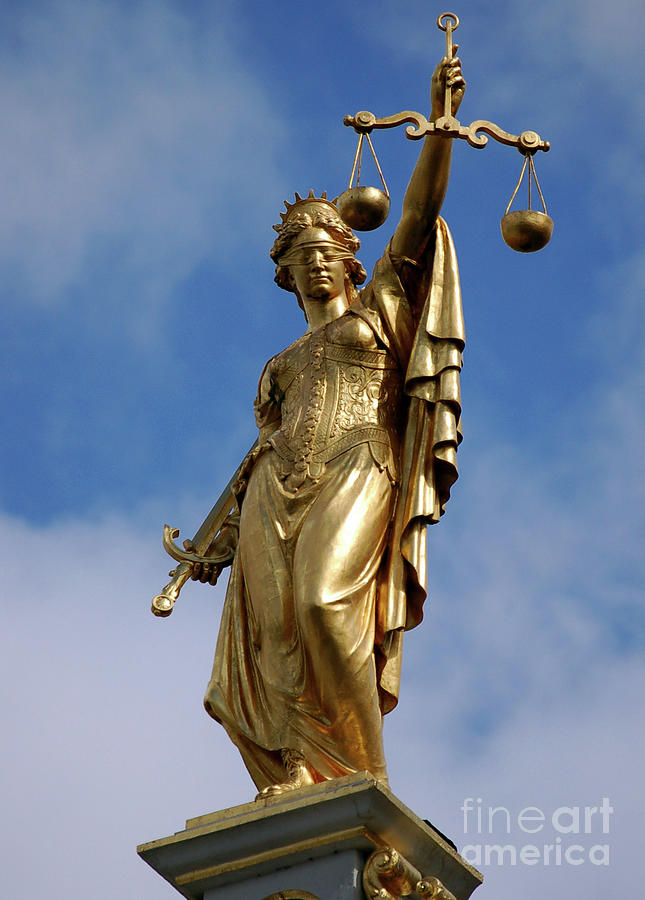This photograph, featuring the logo "Fine Art America" in transparent white text at the bottom right, captures an elegant bronze statue of Lady Justice against a vivid blue sky filled with fluffy white clouds. The statue, which appears to glow in bright bronze and gold hues, stands prominently on a platform. Lady Justice is depicted with a blindfold across her eyes and a crown atop her head. She is intricately detailed, wearing a corset with a long, flowing skirt sculpted to look as if it is billowing in the wind. Over her left arm, which holds the symbolic scales of justice high, she has a flowing cape that cascades down to her feet. In her right hand, she grips a sword that points upwards toward her. This striking image, possibly created for a magazine cover, evokes the classical depiction of justice seen in courtrooms across the United States.